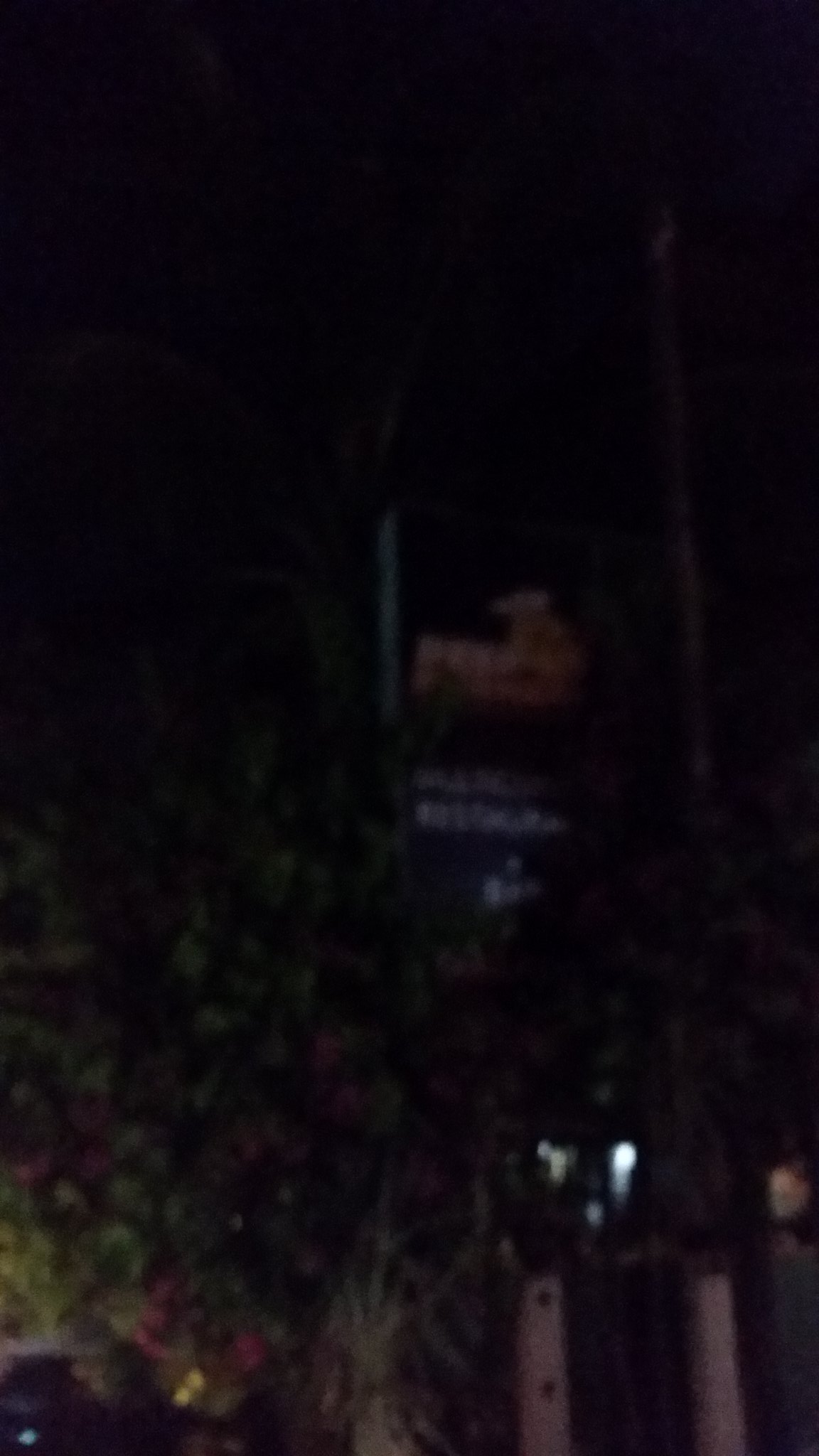This nighttime outdoor photograph features several distinct yet somewhat obscured elements due to the image's low quality. In the bottom right corner, white posts emerge from the ground, partially illuminated by light seeping through an opening—possibly a doorway or window, though the specific source is indiscernible. The bottom left corner showcases green foliage interspersed with pink and purple flowers, adding a touch of color to the scene. Positioned centrally, two signs draw attention despite their blurriness; the upper sign depicts a yellowish figure donning what appears to be a white chef's hat, while the lower, blue sign provides information in white text, though its details remain unreadable.